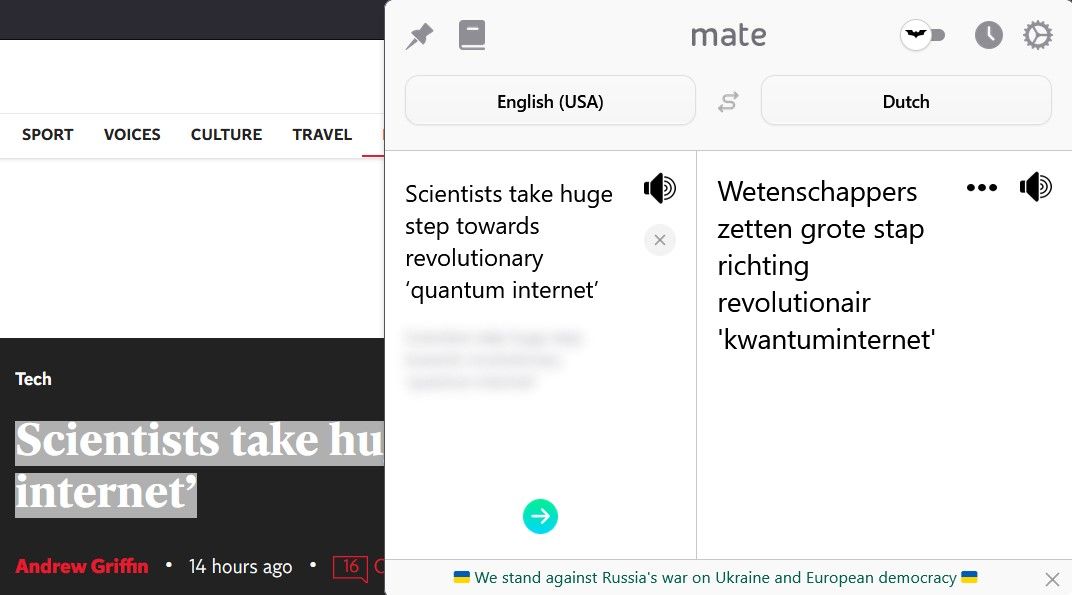This image shows a screenshot of a partially visible web page overlaid with a pop-up window. The underlying web page has a black border and features a white section with tabs labeled "Sport," "Voices," "Culture," and "Travel." A part of the page is visible with text in black reading "Tech" and a partial title starting with "Scientist's Take." It's authored by Andrew Griffin, and the article appears to have been published 14 hours ago.

In the foreground, the pop-up window contains several icons at the top – a pen icon, a book icon, and in the center, the word "Mate." Additional icons include a bird or bat-shaped button, a clock icon, and a settings wheel icon. Below these icons, there are two language selection boxes: the left one displays "English, USA," and the right one shows "Dutch."

The pop-up is divided in half. The left side displays an article headline: "Scientists Take Huge Steps Toward a Revolutionary Quantum Internet," accompanied by a sound icon that is turned on and a closeout square. The right side of the pop-up presents a headline in Dutch: "Wittgenstopper's Zettelgrut Stop Richting Revolutionaire 'Quantum Internet'," followed by ellipses and a sound logo that is also turned on.

At the very bottom of the pop-up, there is a statement: "We Stand Against Russia's War on Ukraine and European Democracy," next to a Ukraine flag and another closeout square.